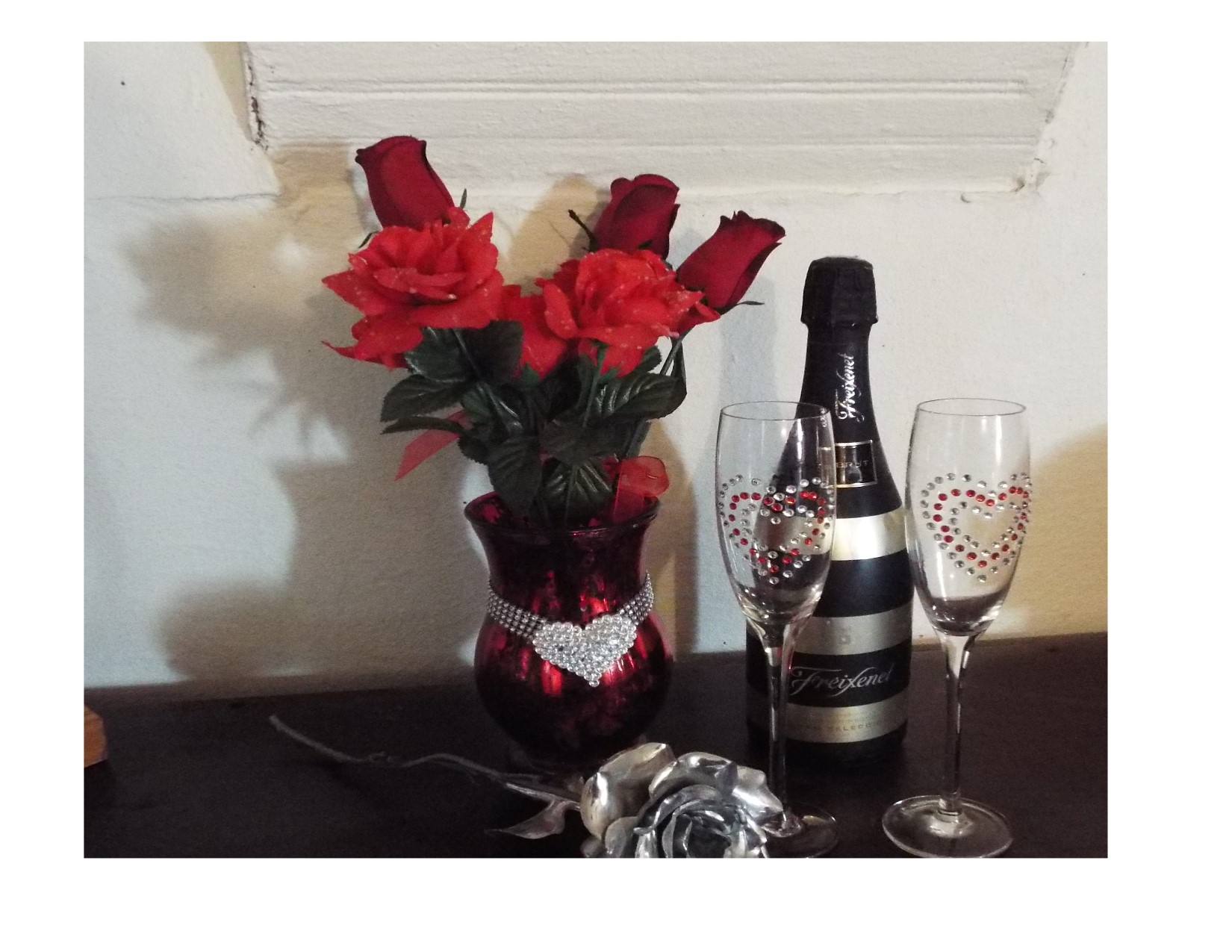This photograph captures a romantic setup, likely intended for an anniversary or Valentine's Day celebration. At the center of the scene is a vibrant, metallic red vase adorned with a silver heart charm and a ribbon embellished with cubic zirconium diamonds. Inside the vase are approximately five short-stemmed red roses, some in full bloom and glistening with water droplets, while others are still in bud. Flanking the vase on the table are two slender, clear wine or champagne goblets, each decorated with red and silver sequins forming heart shapes. A small, unopened bottle of champagne sits nearby, its label indistinguishable but featuring silver metallic stripes. Adding a unique touch to the romantic tableau is a metallic, spray-painted silver or steel rose lying on the dark wooden table or credenza, all set against a plain white wall. The shadows of the objects cast prominently against the wall, enhancing the intimate atmosphere of the photo.